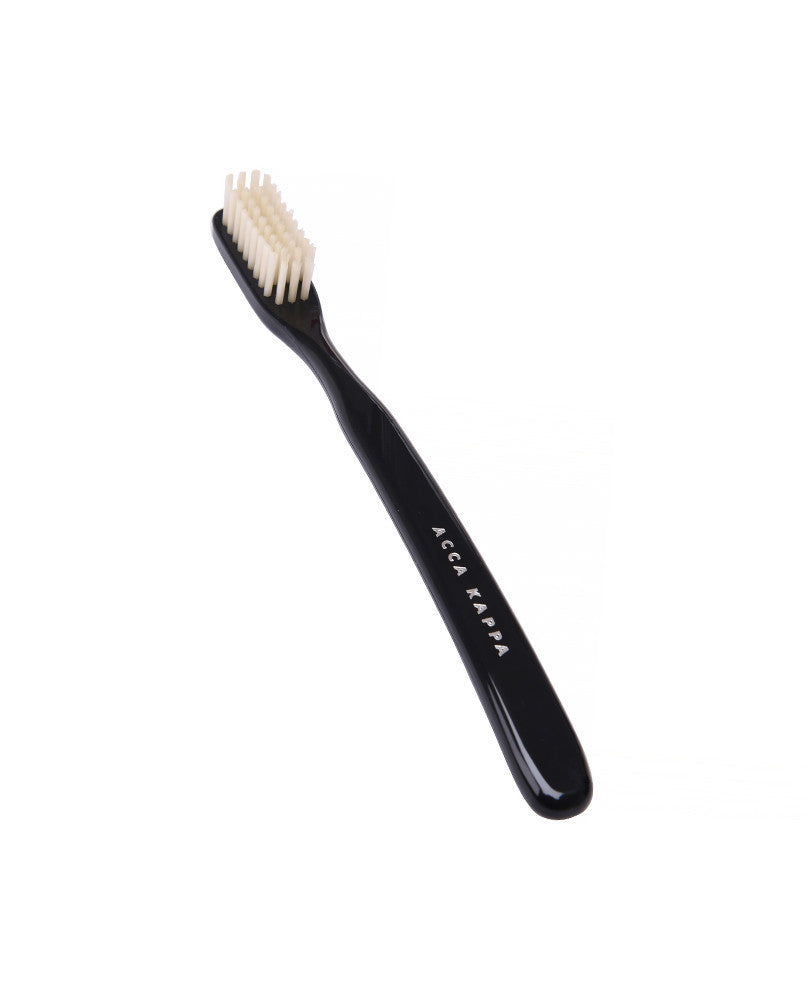The image features a sleek, black, kid-sized toothbrush prominently displayed against a pristine white background. The handle, which curves gently towards the bottom, is adorned with silver-colored text that reads "Acca Kappa" in capital letters, suggesting it might be the brand name. The toothbrush has soft-looking, white bristles, making it suitable for gentle brushing. The light subtly reflects off the handle, giving it a polished and clean appearance. This minimalist composition, with its sharp focus and lack of distractions, makes it ideal for an advertisement, capturing the elegant simplicity and essential details of the toothbrush.